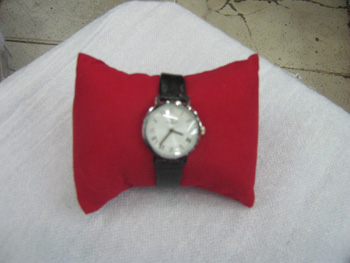This photograph captures a wristwatch precisely reading 3:36. The image is slightly out of focus, making some details a bit challenging to discern. The wristwatch features a pristine white face adorned with black hour and minute hands, and the numbers are elegantly presented in Roman numerals. The band is a sleek black, and the watch is showcased wrapped around a small, red, felt-like pillow. This red pillow rests atop a piece of white fabric, with a tiled floor subtly visible in the background.